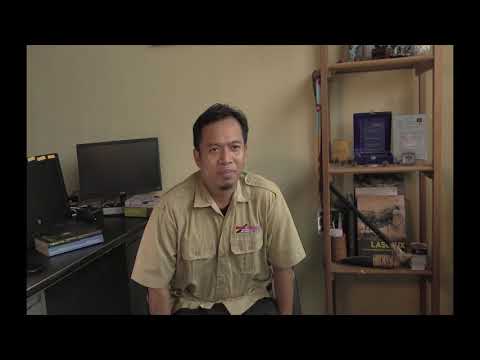The photograph features a middle-aged Asian man seated in an office, wearing a tan short-sleeved worker's shirt with a logo above one of the pockets and a dark shirt underneath. He has black hair, a slight goatee, and a serious expression as he looks at the camera. Behind him, the wall is painted yellow. On the left side of the image, there is a stone desk with two black Dell computer monitors and several books scattered around. To his right is a tall, wooden bookshelf containing books and various decorations. The man has both hands resting on the base of his chair, appearing to be in a neutral state, neither smiling nor frowning.